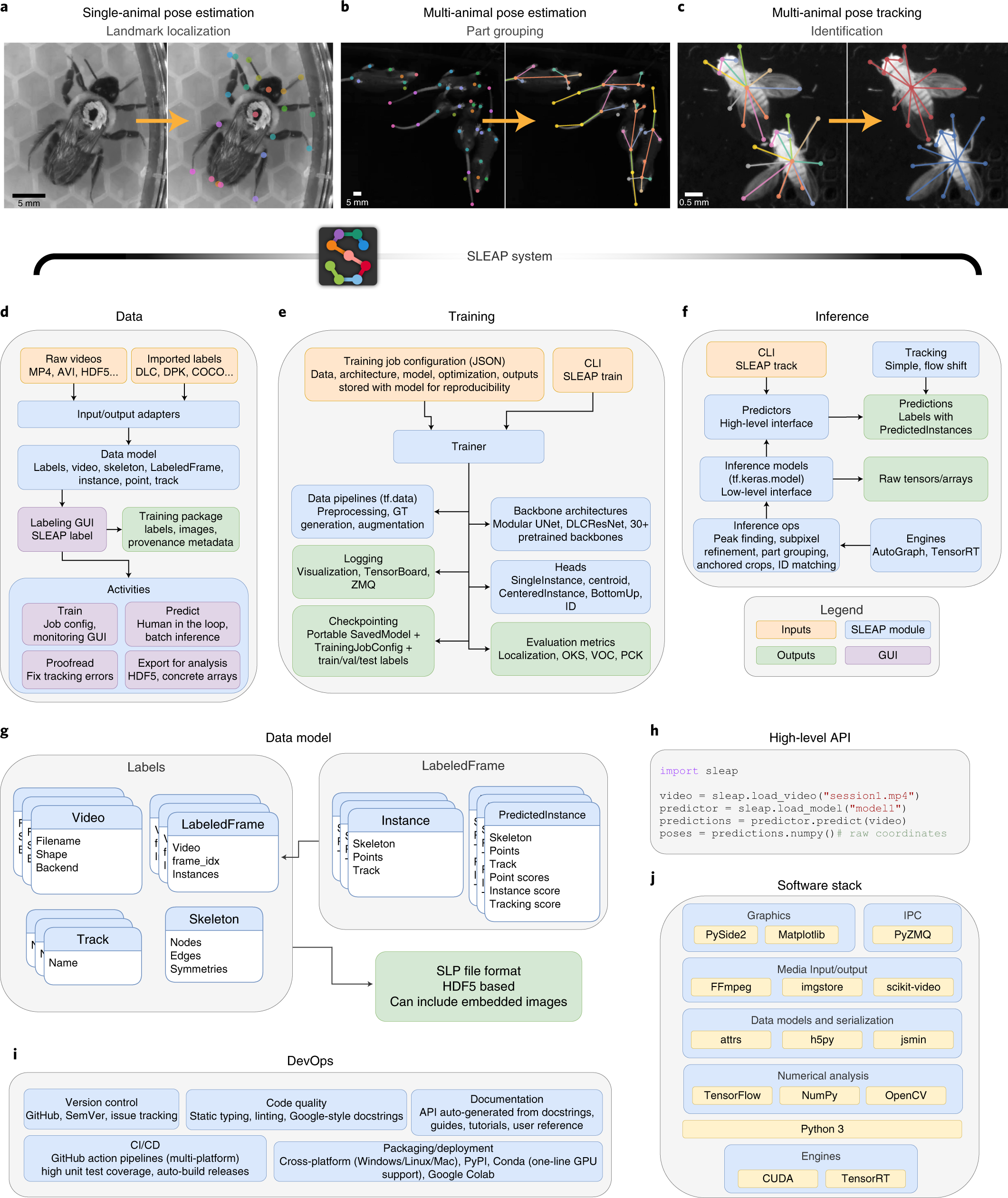This is a detailed page from an educational biology book or research study focused on insects, specifically roaches. At the top of the page are three black-and-white images, labeled from left to right. The first image is captioned "Landmark Localization," showing two insects in a dish. The second, labeled "Part Grouping," features two black images filled with various colored arrows (green, blue, purple, pink), indicating the positioning of different parts. The third image, titled "Multi-Animal Pose Tracking," displays an x-ray of four roaches, two on the left and two on the right, with colored arrows (red, blue, green, and yellow) tracking their movement. Below these images, there's a detailed table of contents arranged into three columns: data, training, and inference. This section mentions tools and concepts like single animal pose estimation, multi-animal pose estimation, the SLEAP system, and multiple animal pose tracking. Additional technical details include high-low API, software stack, and DevOps, organized in a flow-chart style with numerous colored boxes. The page hosts a wealth of scientific information regarding roach studies, showcasing different methodologies for tracking and analyzing their behavior and movement.